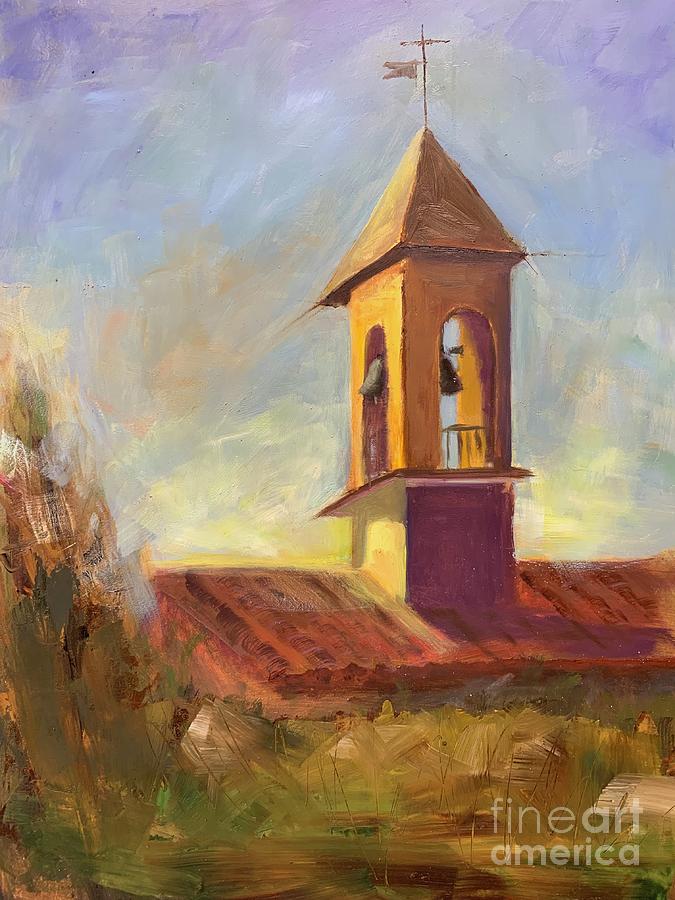This painting, an evocative piece bearing the watermark "Fine Art America" at the bottom right, captures the serene setting of a church and its bell tower. The focus rests on a prominent yellow bell tower situated at the center of a red-roofed building. At the top of this tower, a flag flutters in the clear blue sky, indicating a gentle breeze. The painting displays two church bells, one seemingly in mid-ring. The brush strokes are broad and impressionistic, drawing attention to the bells and the tower while lending a captivating texture to the depiction. A hint of green in the foreground suggests foliage surrounding the church. To the left, a silhouette resembling a scarecrow subtly blends into the composition. The artwork's background melds blues, whites, and subtle afternoon light hues, implying a tranquil late afternoon setting.